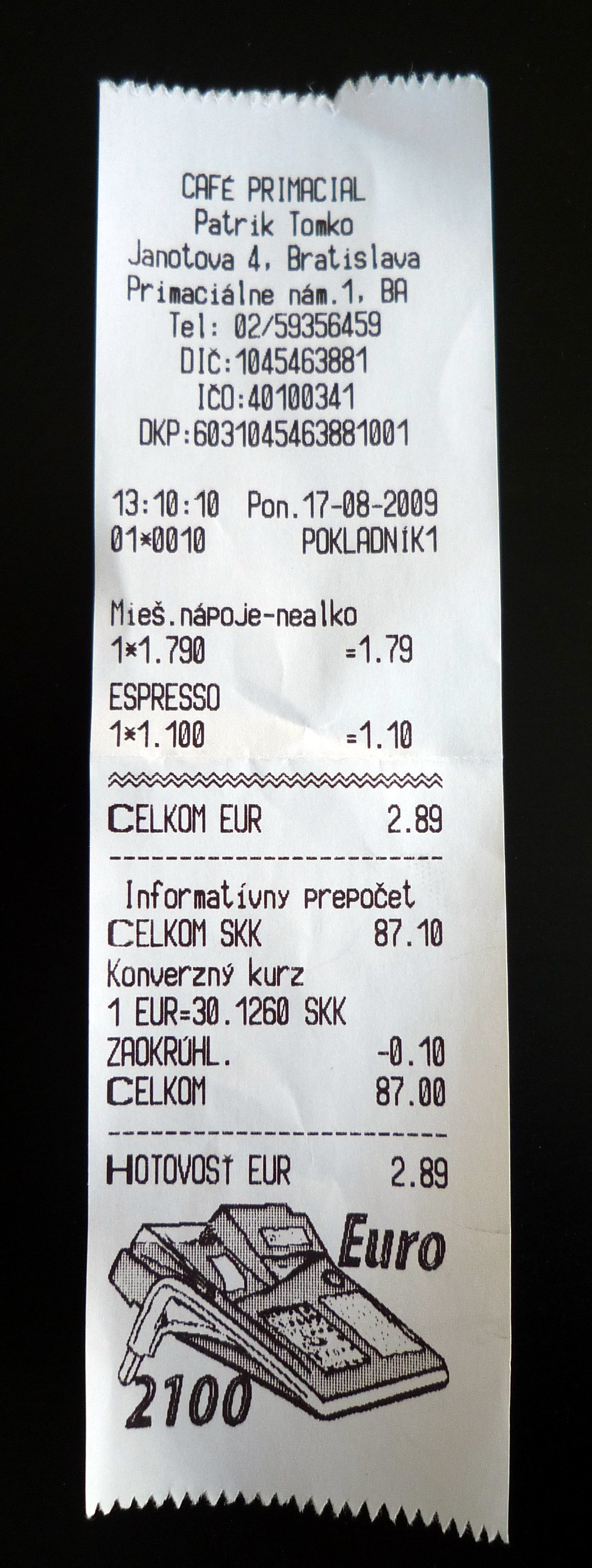A detailed image caption could be formulated as follows:

"This image depicts a long, narrow white receipt from Café Prémiciel, a café located in Bratislava. The receipt is printed in Slovak, the official language of Slovakia. It lists an espresso priced at €1.10 and another item costing €1.79, bringing the total amount to €2.89. At the bottom of the receipt, there is an unusual drawing that appears to be a partial sketch of a stadium or another similarly structured building, adding a unique touch to this everyday document."